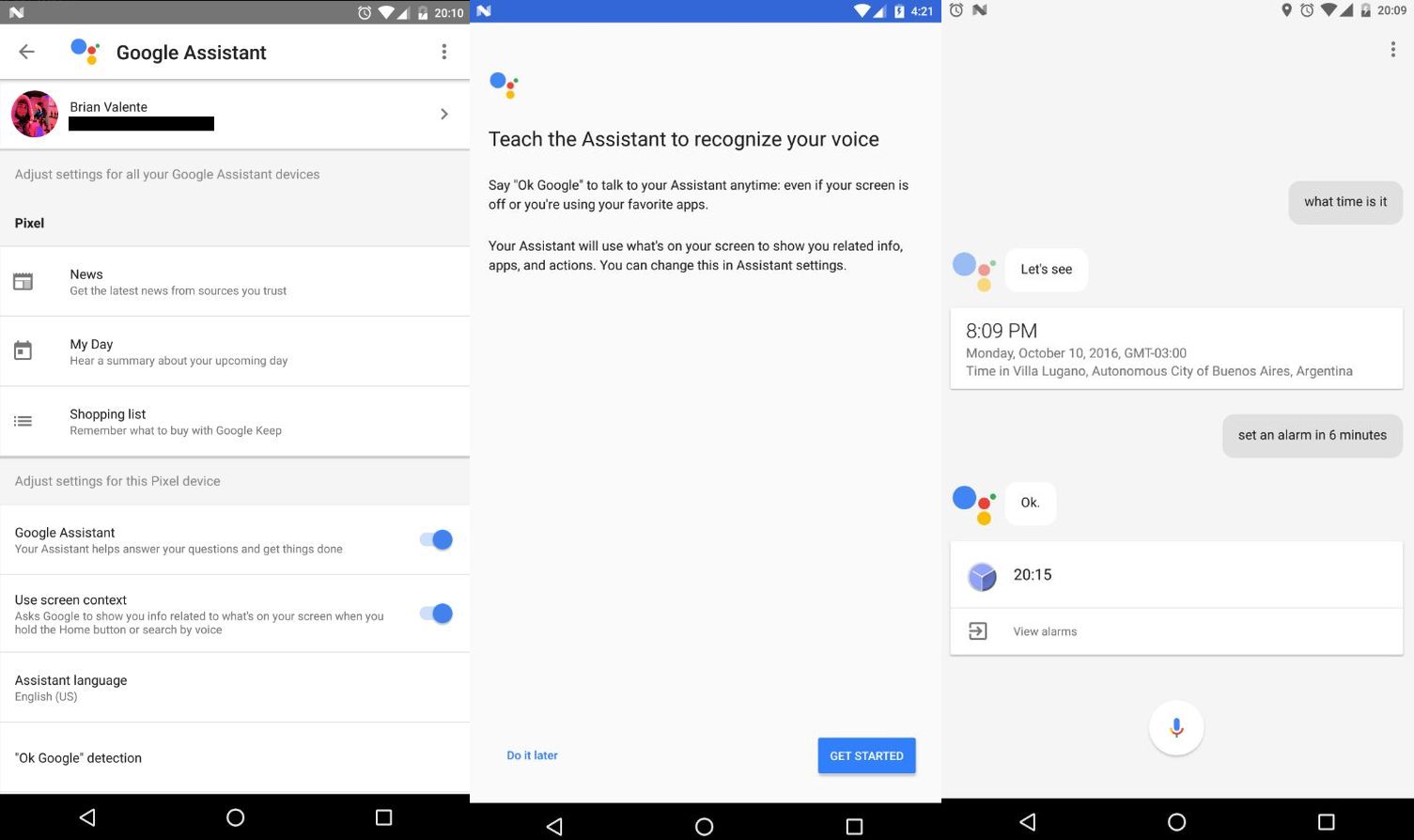Screenshot Collage of Google Assistant Interface and Features

This image showcases a collage of three side-by-side screenshots from Google Assistant on a smartphone. Each screenshot provides a glimpse into different aspects and functionalities of the Assistant interface.

1. **First Screenshot (Left)**:
   - **Header**: "Google Assistant"
   - **User Information**: "Brian Valente"
   - **Options**: Items listed include "Pixel," "News," "My Day," and "Shopping List."
   - **Settings Section**: "Google Assistant in Screen Context" with slider buttons, currently toggled on.
   - **Languages**: "Assistant Language" is set to "English."
   - **Voice Activation**: "OK, Google Detection" setting is visible.

2. **Second Screenshot (Center)**:
   - **Header**: Blue banner with the text "Teach the Assistant to Recognize Your Voice."
   - **Instructions**: Below the header, instructs users to say "OK, Google" to engage with the Assistant at any time, even if the screen is off, or while using other apps.
   - **Interactive Elements**: Two buttons at the bottom, "Get Started" on the lower right and "Do it later" on the lower left.

3. **Third Screenshot (Right)**:
   - **Query and Response**: The user asks, "What time is it?" leading to the response: "8:09 PM, Monday, October 10, 2016, time in Villa Lugano, Autonomous City of Buenos Aires, Argentina."
   - **Follow-Up Command**: The user then commands, "Set an alarm for six minutes," to which the Assistant responds with "OK."
   - **Timestamp**: An additional timestamp noted as "2015" is also present.
   - **Navigation & Status**: Black navigation menu bar at the bottom and status icons, including battery and connectivity indicators, visible on the top of each screenshot.

This collage effectively highlights the range of Google Assistant features, from personalized settings and voice recognition training to real-time queries and commands.